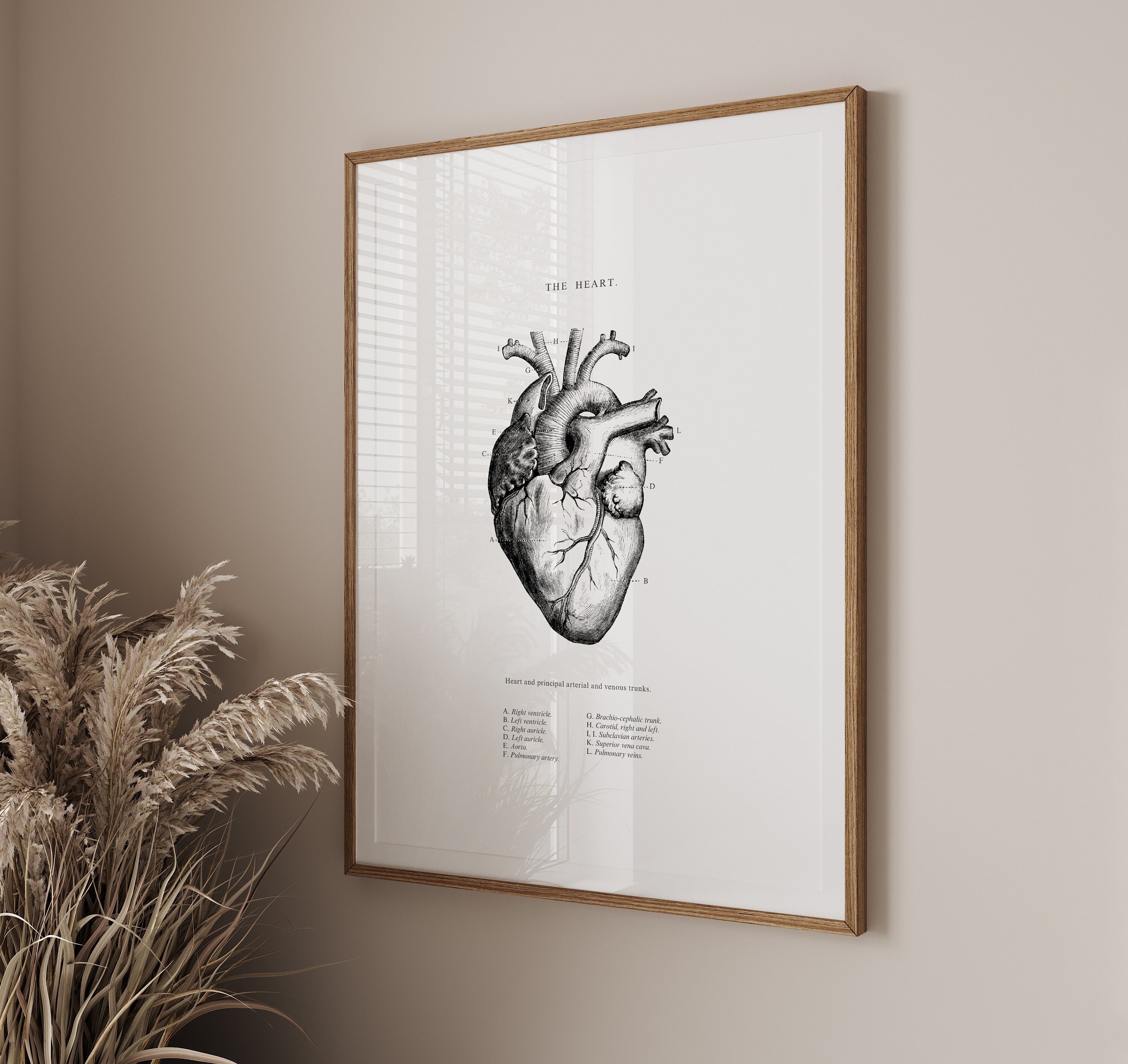The image captures a square photograph of a detailed, framed drawing of a human heart, hanging on a light gray wall. The wooden frame is thin and brownish, encasing the black-and-white heart illustration which is centrally positioned on a white background. The anatomical features of the heart are meticulously labeled, with corresponding labels mapped in a legend situated beneath the heart. The frame itself is viewed from a slightly leftward angle, revealing a plant resembling stalks of wheat extending upwards in the bottom left corner of the image. This arrangement suggests a serene, possibly professional indoor environment, such as a doctor's office.